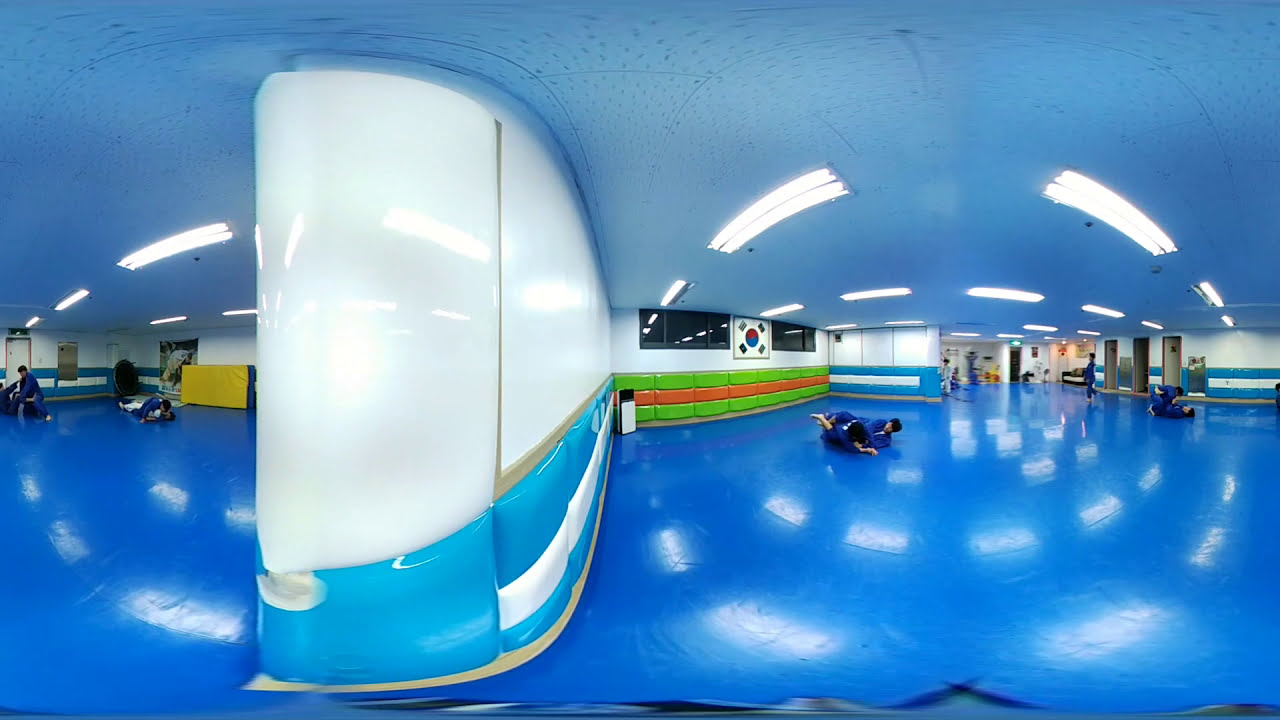This photograph captures a spacious, large indoor hall designed for martial arts practice, possibly judo or karate. The image features two fisheye views, one on each side, providing a broad perspective of the space. The floor is a uniform light blue mat that appears spongy and polished, with overhead lighting reflected off its surface. The high ceiling is also light blue, fitted with bright tube lights that illuminate the entire area.

The hall is divided by a white wall with blue horizontal lines, which splits the room into two distinct sections, creating a two-thirds, one-third visual split. On the right side, which commands more of the focal area, there is a noticeable white wall with a striking neon green lower half separated by a bright orange horizontal line. There are padded sections on the wall featuring green and red stripes, and a South Korean flag is prominently displayed. Windows can be seen to the left and right of the flag.

People in pairs are practicing martial arts on the blue mat, dressed in blue uniforms. Some practitioners are seen wrestling in holds directly on the floor, while others are engaged in various activities farther back in the room, though they appear indistinct due to the distance. The left side of the image, beyond the dividing wall, also shows individuals in blue uniforms, involved in less intense activities compared to the right side. The overall ambiance suggests a dedicated and lively martial arts training environment.